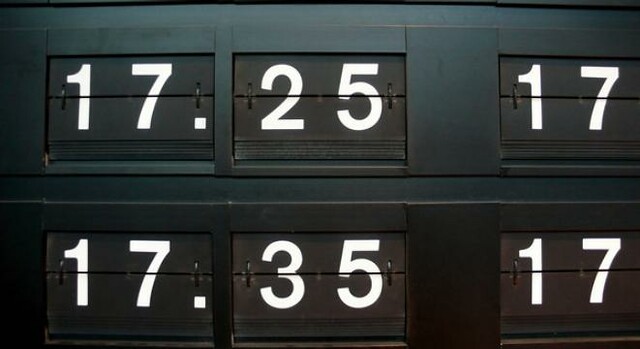The image showcases a grid of numbers displayed on black signs, organized in two rows with three numbers each, all set against a dark blue-black background. 

In the top row, from left to right, the numbers are as follows:
- The first sign on the left displays the number "17".
- The middle sign shows the number "25".
- The rightmost sign also reads "17".

In the bottom row, the sequence of numbers is:
- The first sign on the left displays the number "17".
- The middle sign shows the number "35".
- The rightmost sign again reads "17".

All numbers are in white text on a black background, and the overall composition suggests that the image is taken on a platform or display area, though the close-up nature of the shot focuses solely on the number signs and the dark backdrop.